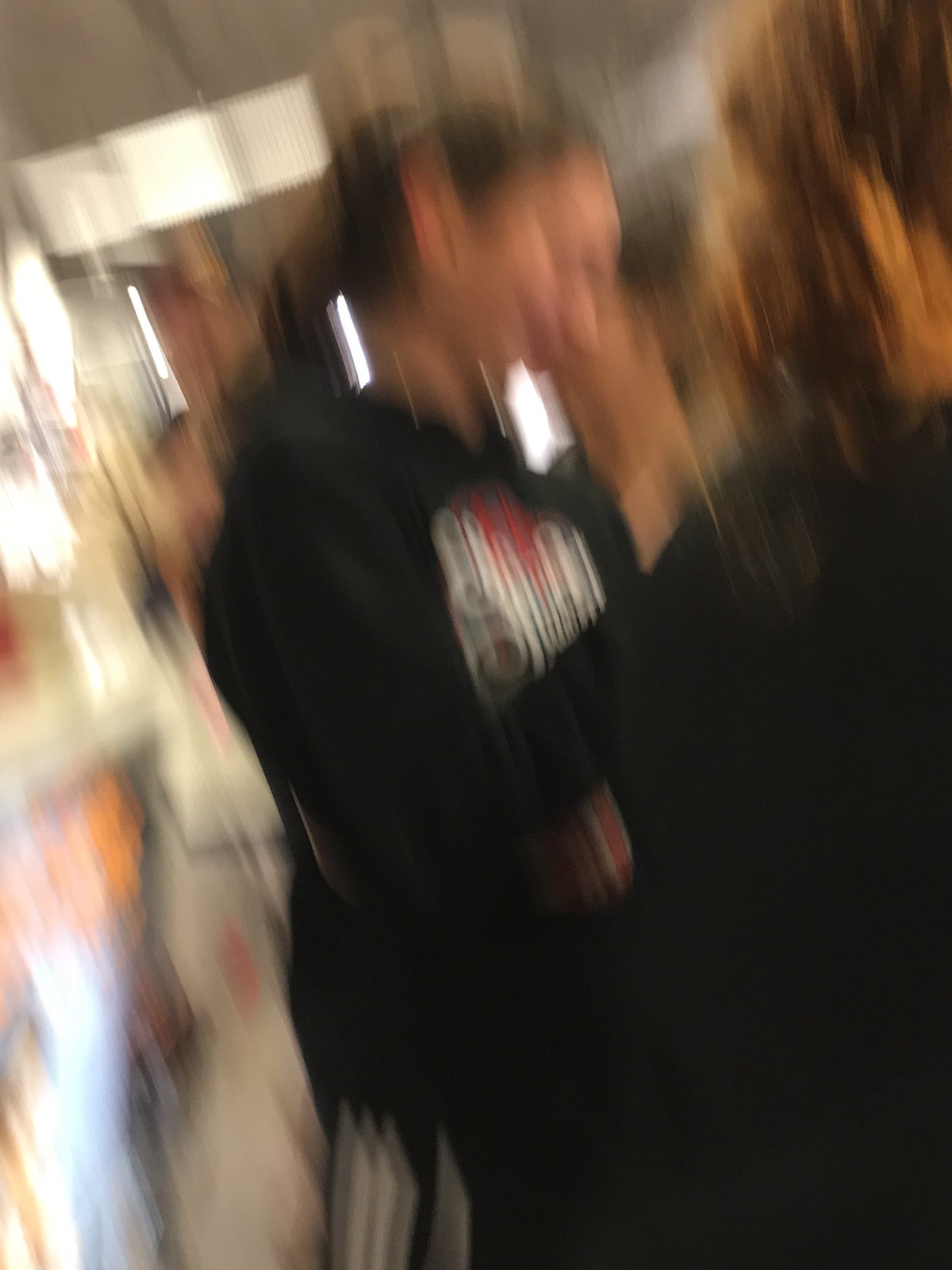An extremely blurry photograph depicting two individuals in what appears to be a store environment. On the right-hand side of the image, there's a person with shoulder-length brown hair, seen from the back, wearing a black shirt or sweater. Dominating the center and left side of the image, a woman with dark hair pulled back behind her ears stands sideways, facing to the right and looking down at something, with her right shoulder visible. She is dressed in a black sweatshirt with a blurred red and white design on the front and black pants with white stripes. The background features indistinct lights and colors, including yellow, orange, and white areas, as well as some faded light pink and brown lights. Fluorescent lights can also be seen on the ceiling, and there are vague shapes of display shelves on the left-hand side, adding to the overall indistinct ambiance of the scene.